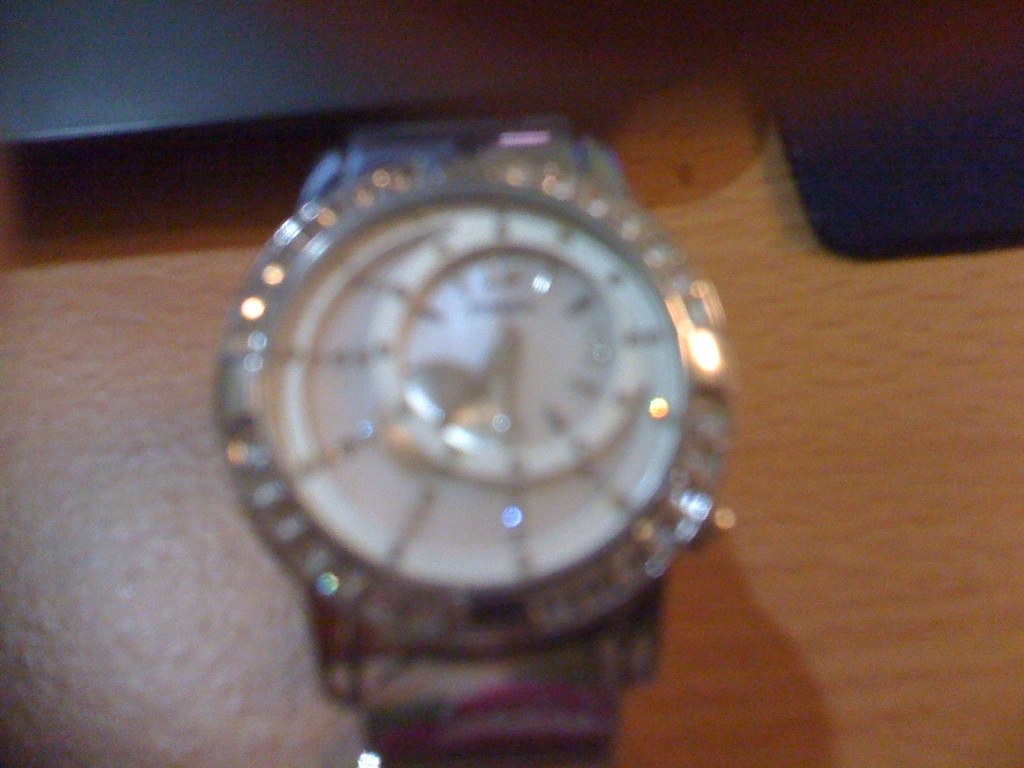The image showcases a silver watch lying on a medium brown wooden desk. The photograph is somewhat blurred, adding a soft-focus effect to the scene. The watch features a white dial and is adorned with sparkling elements around the dial, which might be diamonds or another type of glittering stone. The hands of the watch display the time as 7:30. The watch is equipped with a wide silver band, likely made of metal. In the background, a metallic gray object, possibly a laptop or a similar box, is visible on the desk. To the right side of the image, a bluish pad can also be seen, adding a touch of color to the composition.